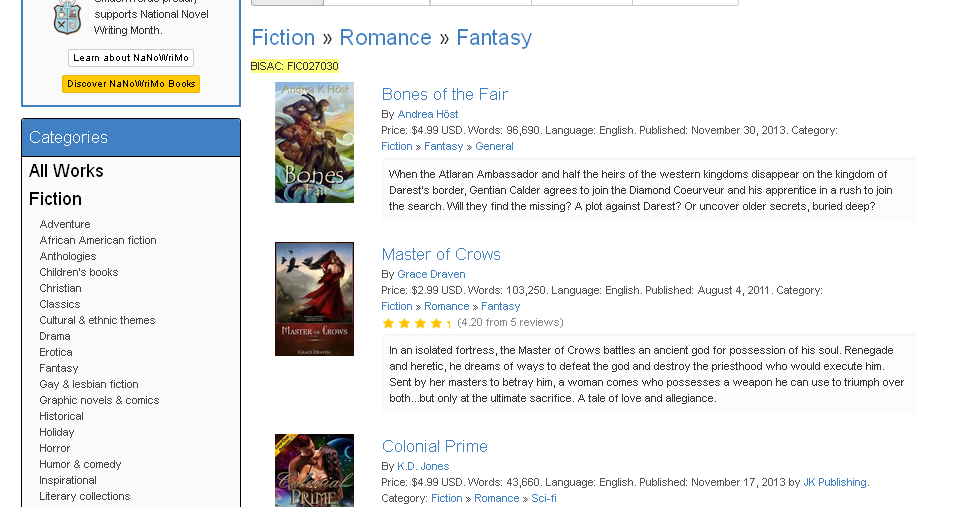This screen capture showcases a website page devoid of any identifying information such as logos or URL bars. On the left side, there are two vertically aligned rectangular sections containing various elements. 

The upper section features a shield-shaped icon and partially visible text that reads "Supports National Novel Writing Month." Beneath this, there are two buttons: a white button with black lettering labeled "Learn About NaNoWriMo," and a yellow button below it that says "Discover NaNoWriMo Books."

The lower section highlights a "Categories" banner in cornflower blue with the text in white, listing various fiction genres under "All Works Fiction."

On the right side of the page, in the upper left corner, there is blue text indicating a navigation path: "Fantasy > Romance > Fantasy." Below this is a yellow-highlighted number labeled "BISAC" followed by a lengthy identifier. Along the left edge of this section are images of book covers accompanied by their titles, prices, genres, and ratings (where applicable):

1. "Bones of Fear" by Andrea Host, priced at $4.99, categorized under Fiction: Fantasy: General.
2. "Master of Crows" by Grace Draven, priced at $2.99, categorized under Fiction: Romance: Fantasy. This book has a rating of 4.20 out of 5 stars.
3. "Colonel Prime" by Katie Jones, priced at $4.99, categorized under Fiction: Romance: Sci-Fi. 

The detailed layout suggests a focus on book listings, particularly those related to NaNoWriMo and various fiction categories.